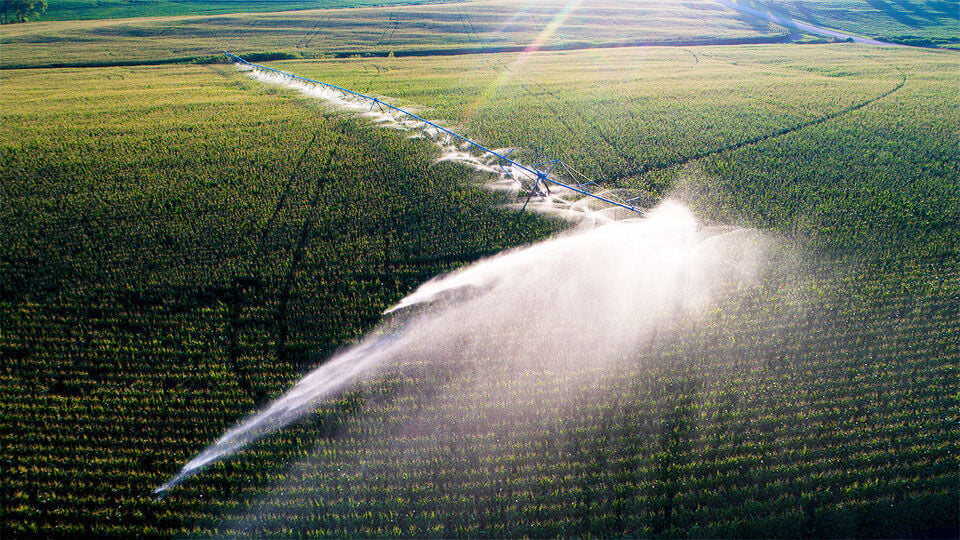An aerial photograph captures a sprawling, irrigated cornfield from several hundred feet above, possibly taken from a drone or airplane. The field is interspersed with a blue metallic sprinkler system, featuring numerous heads that spray water across the verdant crops. These sprinklers are part of an extensive L-shaped irrigation line stretching far into the distance. Tractor tire tracks are visible, marking pathways through the cultivated landscape. On the right side of the image, a two-lane road runs parallel to the cornfield, alongside additional patches of different crops. At the top of the photo, sunlight creates a subtle rainbow effect, imparting a natural touch to the otherwise agrarian scene.